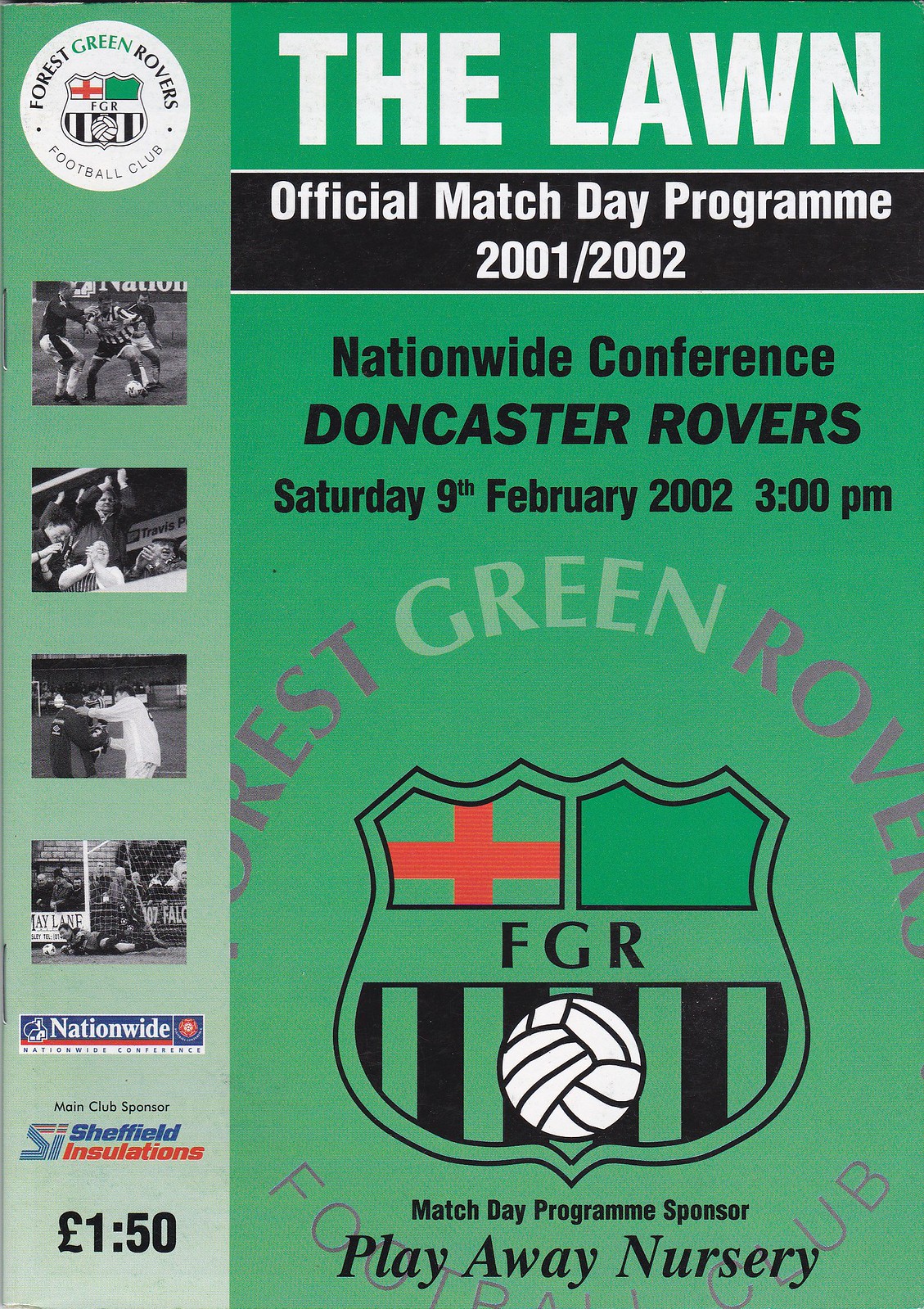This is the cover of an official match day program for a soccer game, set on a primarily green background. The top left features a circular logo with the text "Forest Green Rovers Football Club" in black and green, along with a red flag. Across the top middle of the cover, "THE LAWN" is prominently displayed in all-capital white letters on green. Directly beneath this, on a black banner with white text, it reads "Official Match Day Program 2001-2002". Further down, additional details are presented in black text on a green background, stating "Nationwide Conference Doncaster Rovers Saturday 9th February 2002 3 p.m." The bottom of the cover showcases a logo shaped like a shield containing a soccer ball, sections of green, and a red cross. Directly beneath, "Match Day Program Sponsor Playaway Nursery" is mentioned. The left side of the cover features four rectangular black-and-white photographs showing players and fans, with additional sponsors listed: Nationwide and Sheffield Insulations. At the very bottom, the price of the program is marked as "1 pound 1.50". The cover includes a rich array of colors—green, white, light green, red, black, tan, gray, and blue—adding to its vibrant appeal.